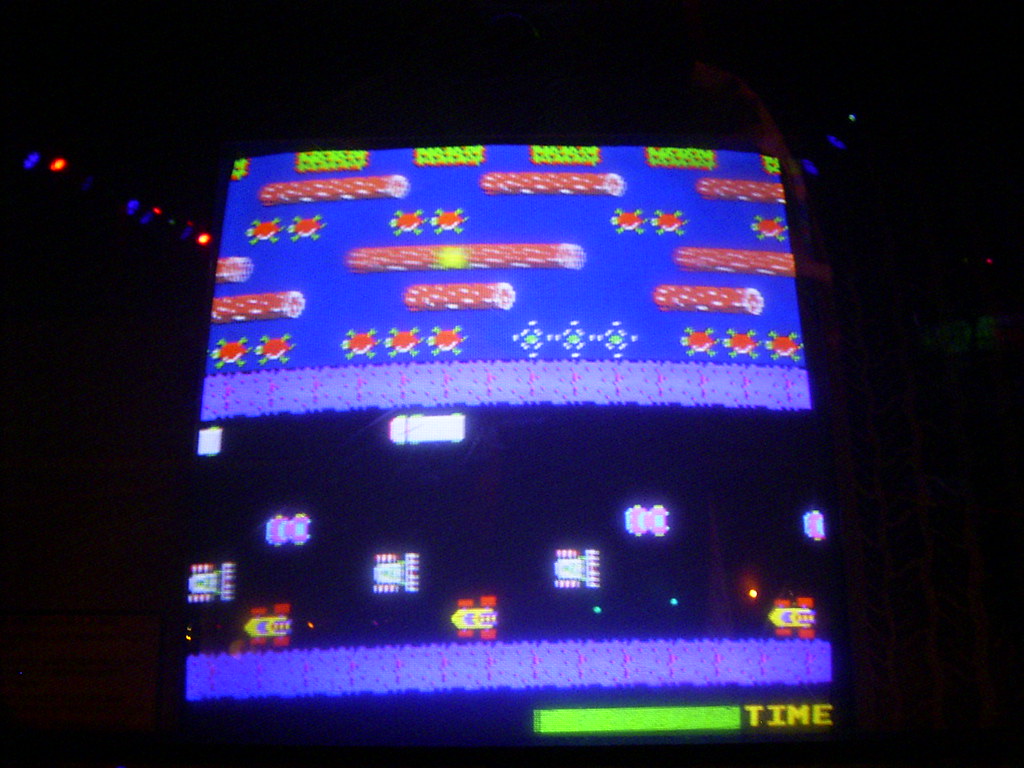The image captures a nostalgic scene from an old arcade game, set against a black background typical of classic CRT screens. The screen features occasional flecks of colorful light, lending an aged, pixelated look. The game layout is divided horizontally into distinct sections. At the bottom right, a green bar labeled "TIME" in yellow indicates it's a timed challenge. Above this, rows of tiny digital racing cars and trucks in various colors—white, yellow, red, and pink—are rendered from a top-down perspective. The vehicles are positioned as if engaged in a race, predominantly on the left side, with a truck on the right. Higher up, the image shifts to logs of varying lengths, interspersed with red elements, possibly floating objects or obstacles. At the very top, yellow squares outlined in red and lime green with more dots create an additional layer of complexity. The game seems to involve navigating these racetrack sections and avoiding obstacles, all within a limited time frame.